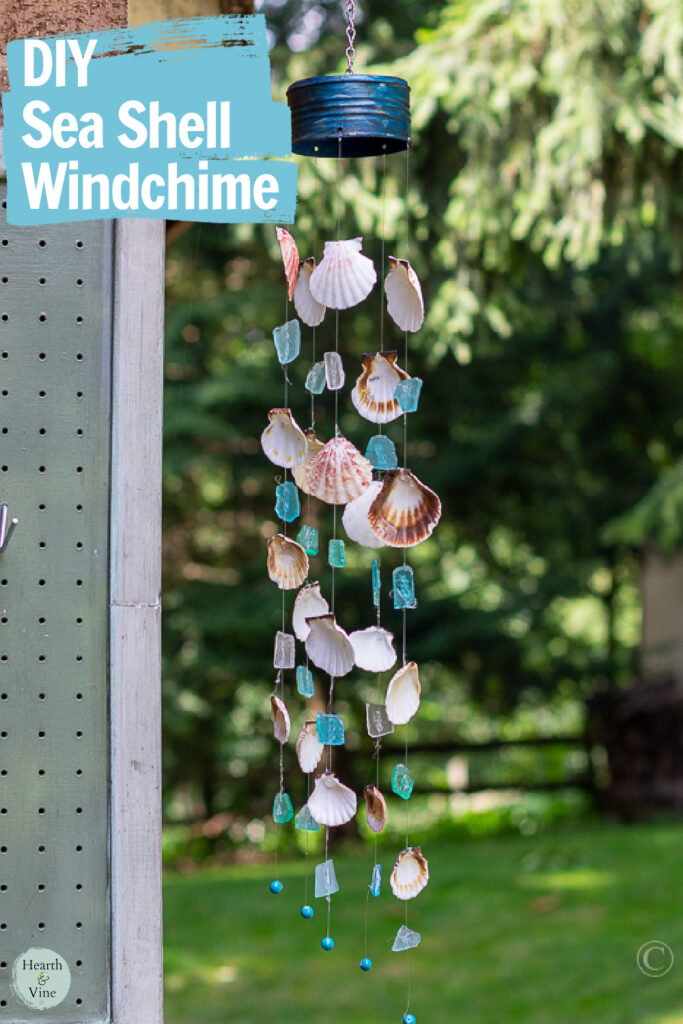The image features a DIY seashell wind chime hanging centrally. The wind chime is suspended from a brown metal chain attached to a cap-shaped, black metallic head. Five strings descend from the head, each adorned with an assortment of seashells in shades of brown, pink, and red, interspersed with blue crystals. To the left of the image is a gray wooden wall with tiny black holes and a light gray wooden edge. The background is an outdoor setting with blurry trees and grasses illuminated by sunlight. The top left of the image displays the text "DIY Seashell Wind Chime" in white ink against a blue backdrop.